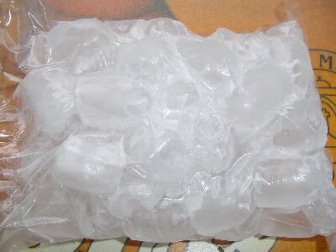A clear plastic bag filled with large, tightly packed ice cubes dominates the image, stretching horizontally across most of the photo with the bottom right corner just barely cut off. The edges of the bag are visible, especially on the left side where the material appears bunched together. The ice cubes are somewhat frosted, and the bag clings tightly around them, indicating that the air has been mostly removed, causing the ice cubes to stick together, likely from partial melting and refreezing. There is some condensation or frost on the bag. This bag of ice is resting on a brownish-orangish background, which appears to be a pizza box, with some black designs and white print visible towards the back right. The letter "M" can be seen in the background, adding a stark contrast to the overall image.